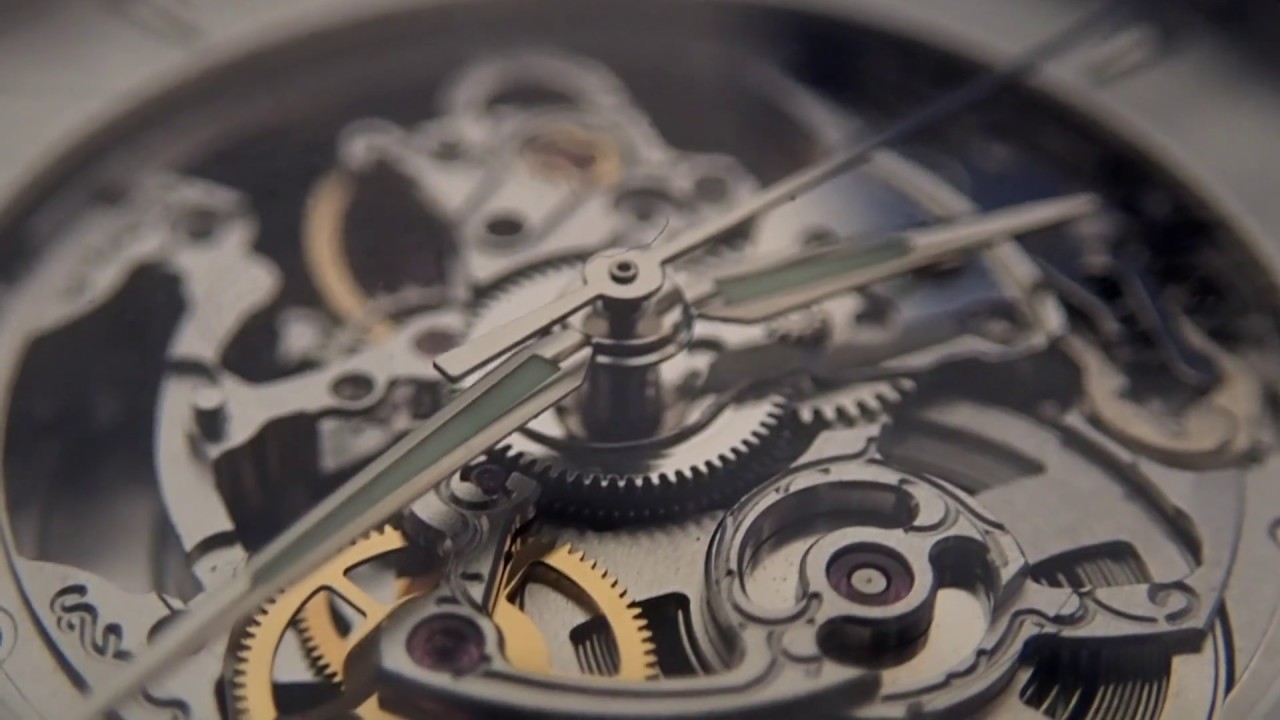The close-up image reveals the intricate internals of a clock or watch. Dominating the center are multiple gears, including a prominent brass-colored gear and several dark silver gears that intricately connect to drive the timekeeping mechanism. The clock features three distinct hands: a second hand pointing to the top right, and minute and hour hands with a green center, contributing to the clock's precise functionality. The hour and second hands are aligned towards the top right, while the minute hand points to the bottom left. The background of the image subtly blurs towards the top, accentuating the detailed craftsmanship and the metallic sheen of the components within this mechanical masterpiece.